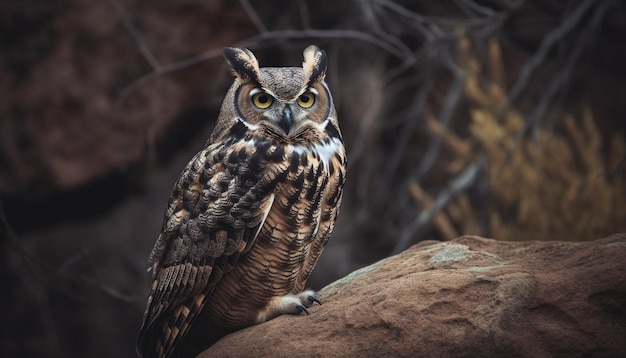This photograph captures a detailed image of an owl perched on a brown rock. The owl is primarily light brown with various shades of brown, black, and cream feathers. It has striking large yellow eyes with very black pupils that almost look starry. White markings above its eyes create an illusion of eyebrows, giving it a stern and intense expression, and a heart-shaped facial outline. The owl has black streaks and dots across its feathered chest, complemented by prominent feather formations above the eyes resembling horns. Its sharp, black beak is forward-facing, adding to its vigilant appearance. The background is blurry, enhancing the focus on the owl. It's surrounded by blurred branches, sticks, and leaves, giving an impression of its natural forest habitat. The lighting suggests a cave-like atmosphere, with light filtering down from above, which adds a touch of mystery to the scene.